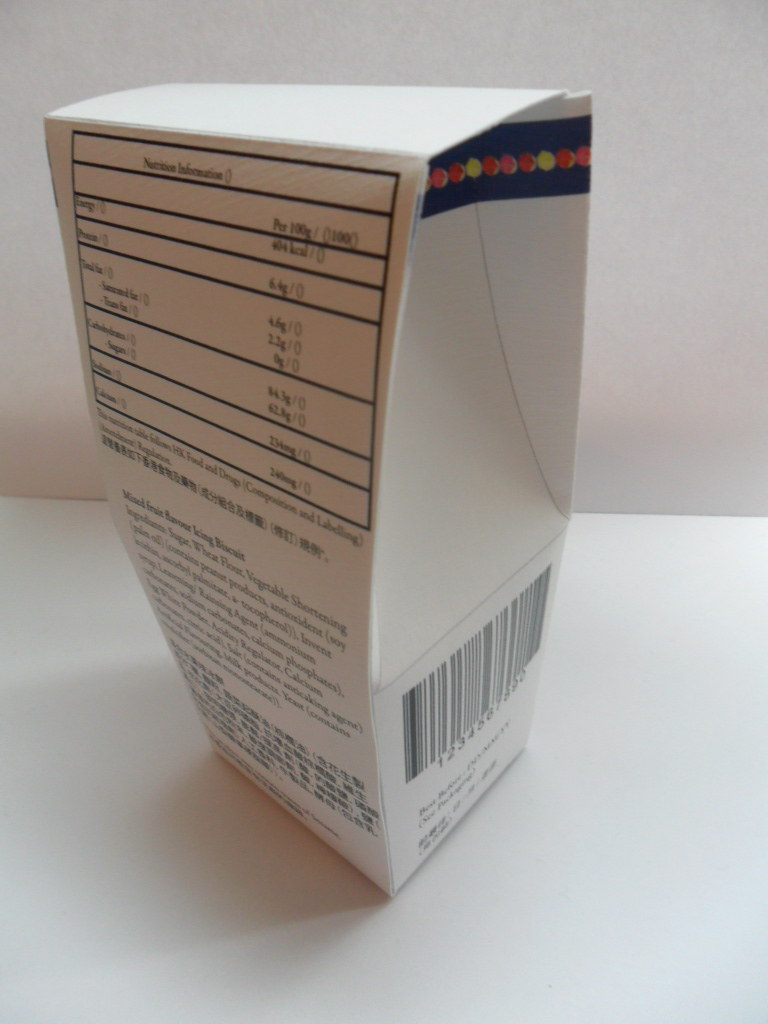The image features an unusual, tall, and elongated food box labeled "Mixed Fruit Flavor Icing Biscuit." The box is primarily white with an eye-catching blue strip adorned with orange, red, yellow, and pink dots on one of its sides, potentially indicating the various fruit flavors of the biscuits inside. Its shape appears to be somewhat indented on the side, making it unique in appearance. 

On the back, the nutritional information is printed, but it's quite difficult to read. Some discernable values include: 
- Energy: 40.4 kcal
- Total Fat: 4.6 grams
- Saturated Fat: 2.2 grams
- Trans Fat: 0 grams
- Carbohydrates: 84.3 grams
- Sugars: 62 grams
- Sodium: 234 milligrams
- Calcium: 240 milligrams

The box also mentions regulatory information including "Food and Drugs, Cosmopolitan, and Labeling Regulation" in English, followed by some text in Chinese. The ingredients list includes wheat flour, sugar, vegetable shortening, peanut products, and soy, among others. Additionally, a barcode is present on the side panel.

This product stands out due to its distinctive packaging shape and colorful design elements, even as the specific details and labeling presented in both English and Chinese add to its intrigue.